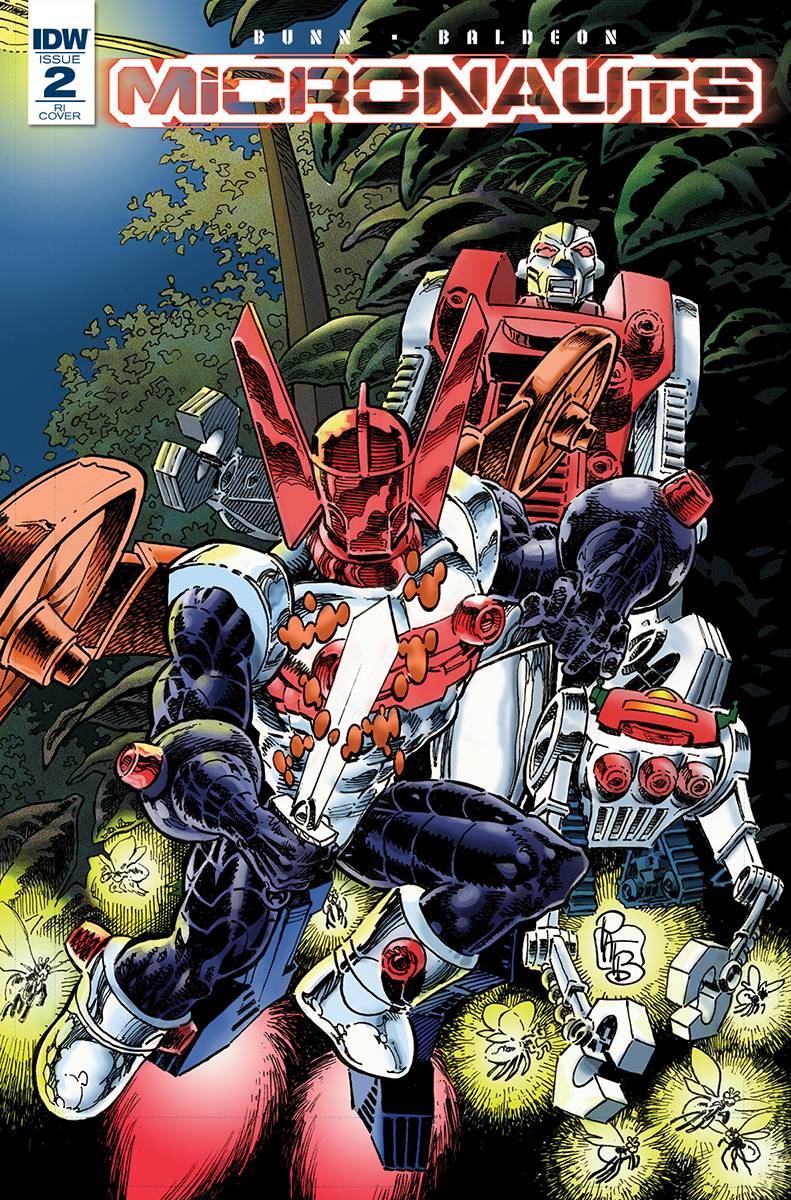This is a detailed depiction of a comic book cover, specifically titled "Bun Baldian: Micronauts," prominently displayed at the top. The words "Micronauts" are highlighted in a striking red and white font. In the upper left corner, it reads "IDW Issue 2 RI Cover" in blue letters against a white background. The main focus of the illustration is a futuristic, robotic figure reminiscent of a Transformer. This intricate machine has a humanoid form with arms, legs, and a large helmet-like shield over its head. Its outfit features a bold color scheme of black, red, and white, with details suggesting space shoes that might even have fire emanating from them. Behind this primary robot, there appears to be another machine-like entity sharing a similar color palette. Additionally, illuminated yellow insects, possibly fireflies, float around them, casting a glowing light. In the backdrop, some trees add depth to the scene, enhancing the sci-fi ambiance.